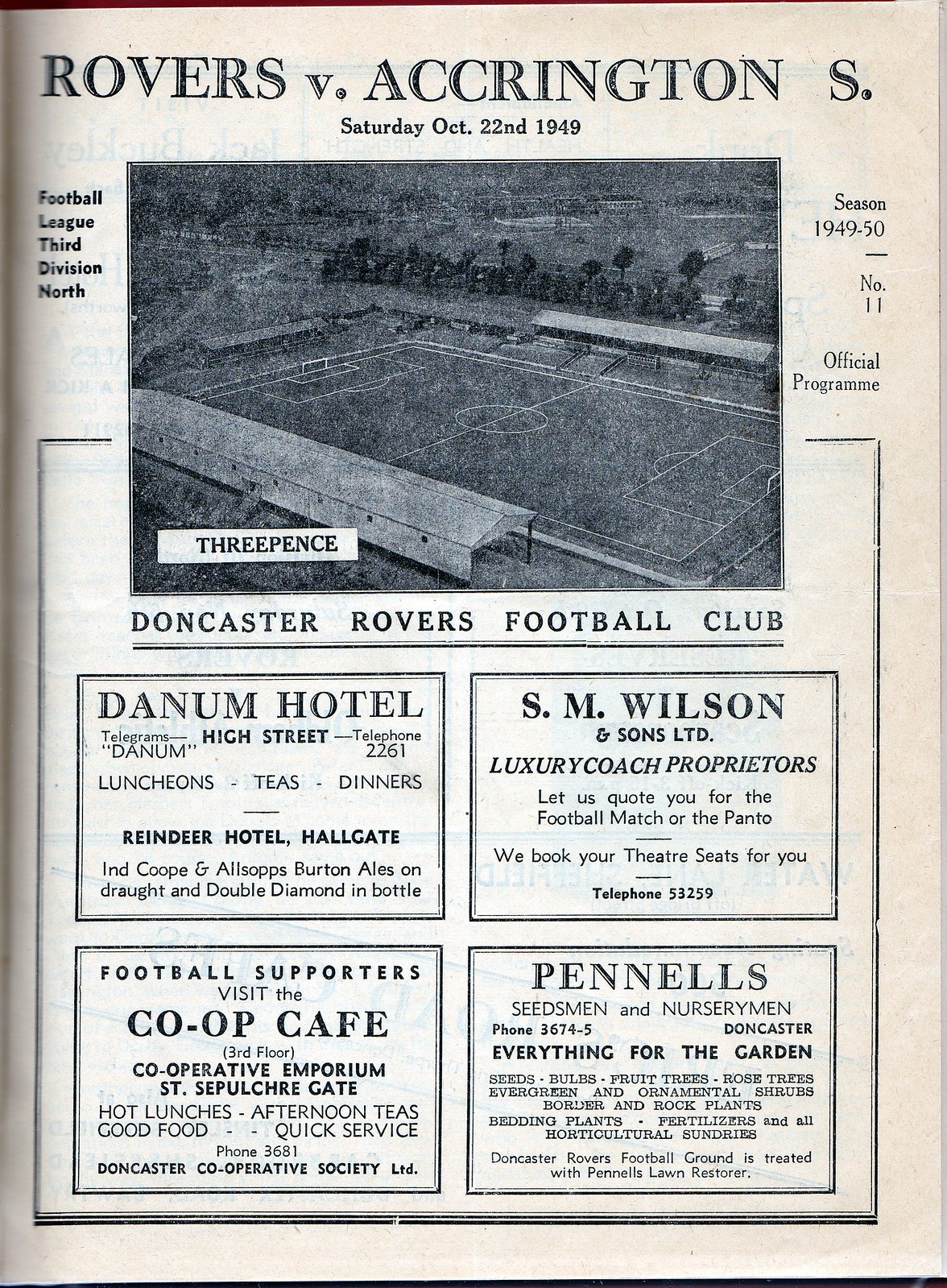The image depicts the front cover of an old rectangular-shaped program from a European football match, specifically for Doncaster Rovers Football Club. The background of the program is off-white, aged with a grayish-blue tint. At the very top, bold black text reads "ROVERS v. ACCRINGTON S." below which it states, "Saturday, October 22nd, 1949." Centrally located is a square, black-and-white aerial photograph of an empty soccer field, suggesting readiness for an upcoming game.

On the left side of the photograph, the text "Football League, 3rd Division North" is printed, and on the right side, it states, "Season 1949-50, No. 11 Official Program." In the lower-left corner of the photograph, there is a white rectangle with the price "3 pence." Below the photograph, the title "Doncaster Rovers Football Club" is underlined and printed in bold.

At the bottom, four advertisements are arranged in a 2x2 grid. The top-left advertisement promotes the "Danum Hotel, High Street," with services like luncheons, teas, dinners, and mentions of "Reindeer Hotel, Hallgate," along with beverages like Burton Ale. The top-right ad is for "S.M. Wilson & Sons Limited, Luxury Coach Proprietors," offering services for football matches and theater bookings, with their contact number being 53259. The bottom-left square advertises the "Co-op Cafe" on the third floor of the Cooperative Emporium, highlighting hot lunches, afternoon teas, good food, quick service, and includes a contact number, 3681. Finally, the bottom-right box advertises "Pennell's Seedsmen and Nurserymen," providing a variety of gardening supplies and stating that the Doncaster Rovers Football Ground is maintained with Pennell's Lawn Restore, with their contact number listed as 3674-5.